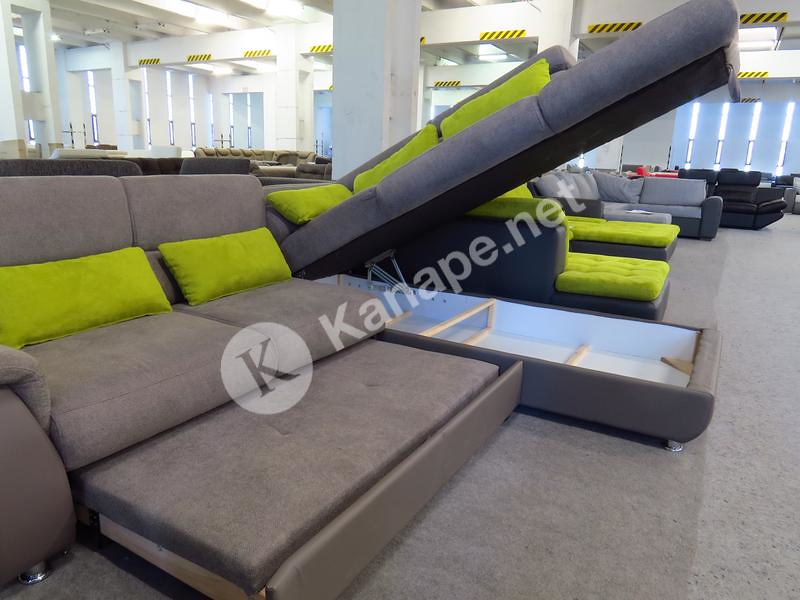This photograph captures the interior of a spacious furniture store, illuminated by bright ceiling lights which highlight several white stone pillars spread throughout the room. Central to the image is a prominent L-shaped sectional couch, predominantly grey in color, featuring lime green rectangular pillows. The sectional includes a multifunctional design, with one of the seats capable of sliding out to create a large footrest. Additionally, the L-section of the couch lifts up to reveal a storage space beneath, supported at an angle by steel bars. In the background, various other couches in shades of gray, black, and light blue are visible, set against large, bright windows with white coverings.